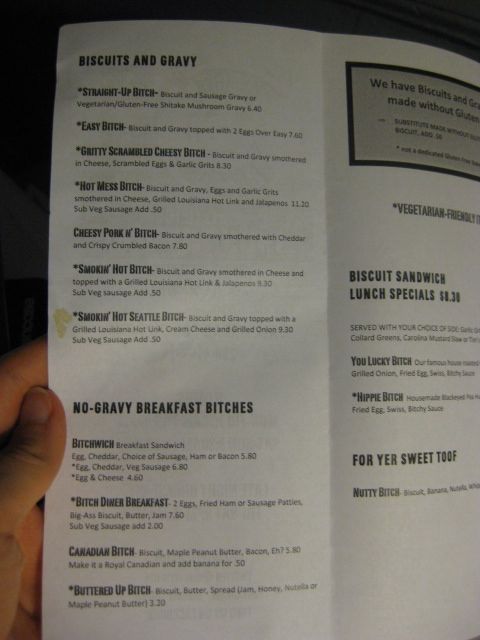This image shows a slightly stained restaurant menu, presented on paper with a noticeable puddle-like stain towards the middle left panel. The menu features a playful and unique naming convention for its dishes, particularly focusing on biscuits and gravy. Under the heading "Straight-up Bitch," diners can choose from:

1. **Biscuit and Sausage Gravy or Vegetarian & Gluten-Free Shiitake Mushroom Gravy** – $6.40
2. **Easy Bitch** – Biscuit and gravy topped with two eggs over easy for $7.60
3. **Gritty Scrambled Cheesy Bitch** – Biscuit and gravy smothered in cheese, scrambled eggs, and garlic grits for $8.30
4. **Hot Mess Bitch** – Biscuit and gravy with eggs, garlic grits, cheese, grilled Louisiana hot link, and jalapenos for $11.30 (vegetarian sausage substitution available for an additional $0.50)
5. **Cheesy Porkin Bitch** – Biscuit and gravy smothered with cheddar and crispy crumbled bacon for $7.80
6. **Smokin Hot Bitch** – Biscuit and gravy smothered in cheese, topped with a grilled Louisiana hot link, and jalapenos for $8.30 (vegetarian sausage substitution available for an additional $0.50)
7. **Smokin Hot Seattle Bitch** – Biscuit and gravy topped with a grilled Louisiana hot link, cream cheese, and grilled onions for $9.30 (vegetarian sausage substitution available for an additional $0.50)

In addition to these, the menu outlines several other categories: "No Gravy Breakfast Bitches," "Biscuit Sandwich Lunch Specials," and offerings "For Your Sweet Tooth." A noteworthy sign at the bottom informs customers that the restaurant also offers biscuits and gravy made without gluten.